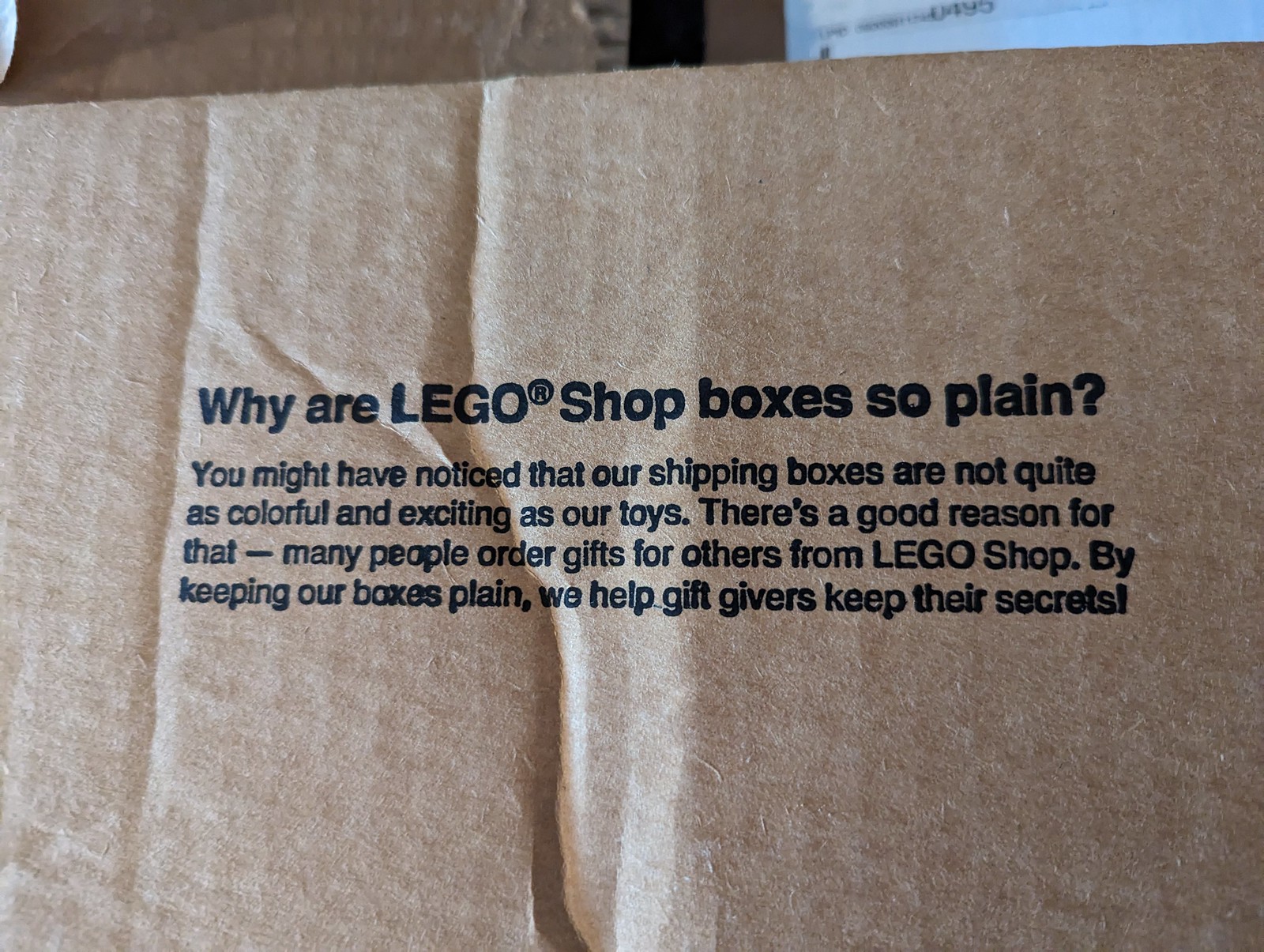This color photograph is a close-up of the flap of a recently opened brown cardboard shipping box from the LEGO shop, showcasing small, bold black printed text. The message reads, "Why are LEGO shop boxes so plain? You might have noticed that our shipping boxes are not quite as colorful and exciting as our toys. There's a good reason for that. Many people order gifts for others from LEGO shop. By keeping our boxes plain, we help gift givers keep their secrets!" The flap, which has a noticeable crease in the middle, is part of a box featuring two other folded-down, torn flaps. A partially visible white shipping label with the characters "UPS 0495" confirms its recent shipment. In the slightly out-of-focus background at the top of the image, you can see another brown box and part of a computer screen, with a glimmer of light on the edge of the box.